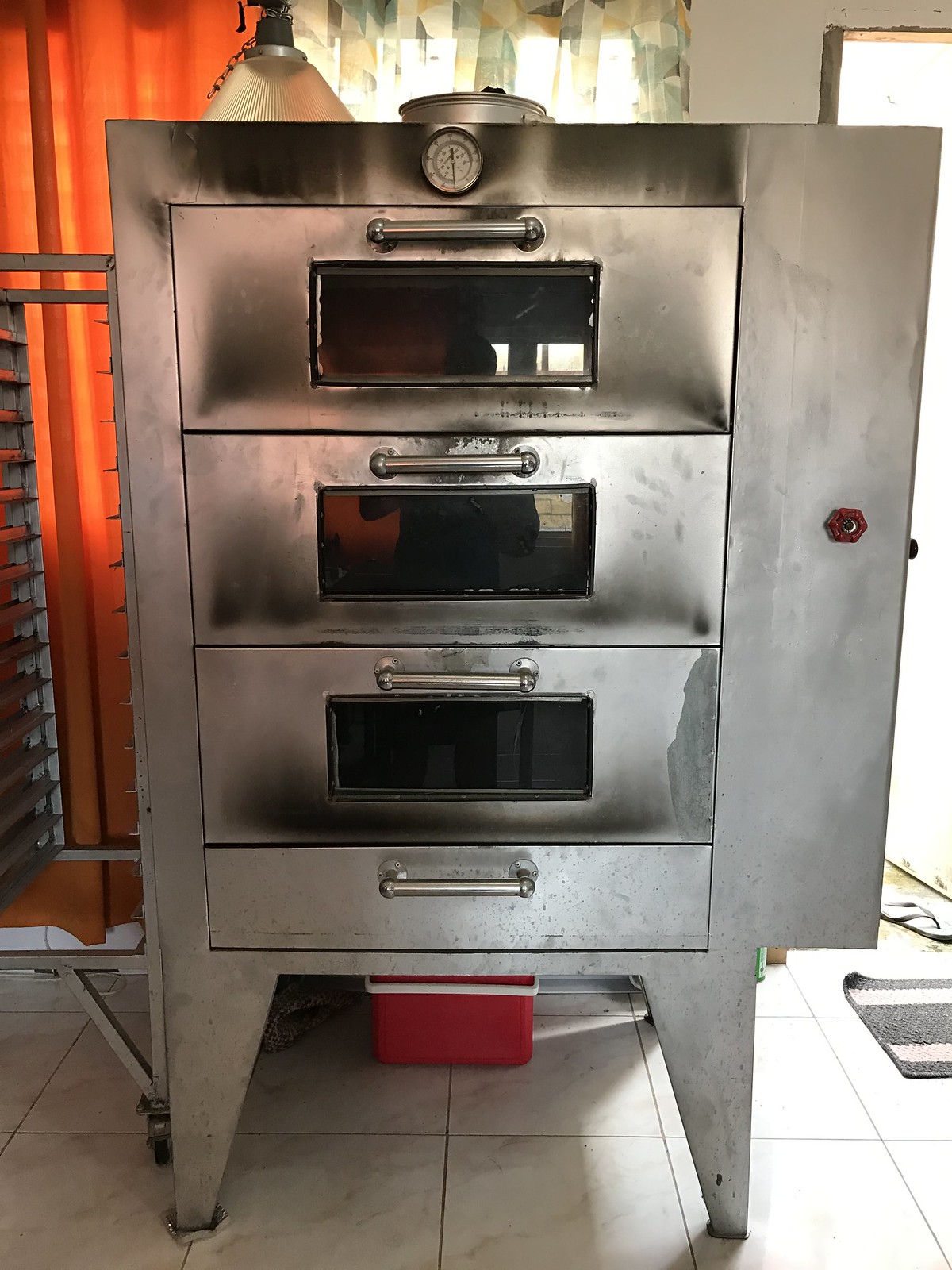The image features a robust, silver pizza oven reminiscent of those found in pizzerias. This large oven, standing approximately five feet tall, has three individual doors, each fitted with rectangular windows for viewing the interior, and is topped with a white-faced temperature gauge at the center. Below these doors is a wider drawer or storage compartment, essential for storing utensils or other items. The oven's face is marked with black soot, indicating frequent use, and even shows a faint handprint. Additionally, there is a red shut-off valve, likely for gas control.

To the right of the oven, a pizza rack is attached for sliding pizzas in and out, and below, a red cooler can be seen resting on a white-tiled floor. Behind the oven, there is a dual-layer curtain setup: a sheer floral-patterned one and a solid orange one, suggesting a somewhat homely or casual setting. A mat and a stray flip-flop near the doorway hint at the familiarity of the place, possibly a home kitchen. The reflection of a man taking the photograph is visible in the oven's glass, providing a candid glimpse into the scene.